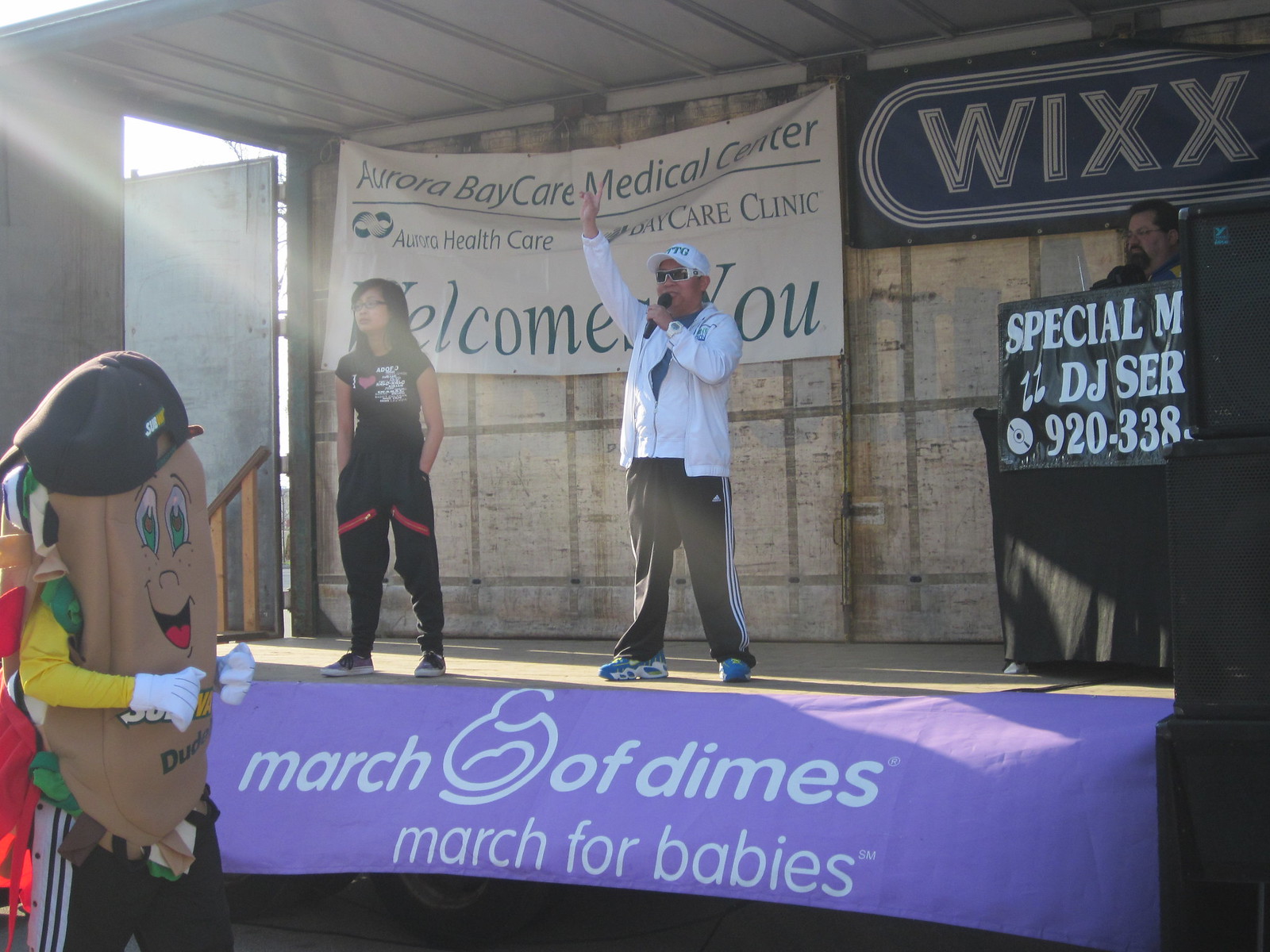A man and a woman are standing on a small stage inside a building, next to an open doorway leading outside with wooden railings descending steps. The woman, dressed in black shirt and pants with red stripes across her thighs, has shoulder-length black hair and looks forward slightly to the right. Beside her, the man, clad in a white coat, white cap, sunglasses, black pants, and blue shoes, raises his right arm while holding a microphone with his left hand. They are backed by a wall with square patterns and an overhead banner that reads "Aurora BayCare Medical Center" and includes the partially visible words "welcomes you." The purple banner draped across the front of the stage displays "March of Dimes, March for Babies."

To the right of the man on stage sits a bearded individual with glasses, short black hair, and black equipment. A sign nearby begins with "special M" and partially reads "DJ SER" and what appears to be a partial phone number "920338." Above him on the wall, another sign reads "WIXX."

On the left side of the image, a person dressed in a mascot outfit resembling a Subway Sandwich, with a black hat and black pants with white stripes, walks towards the right.